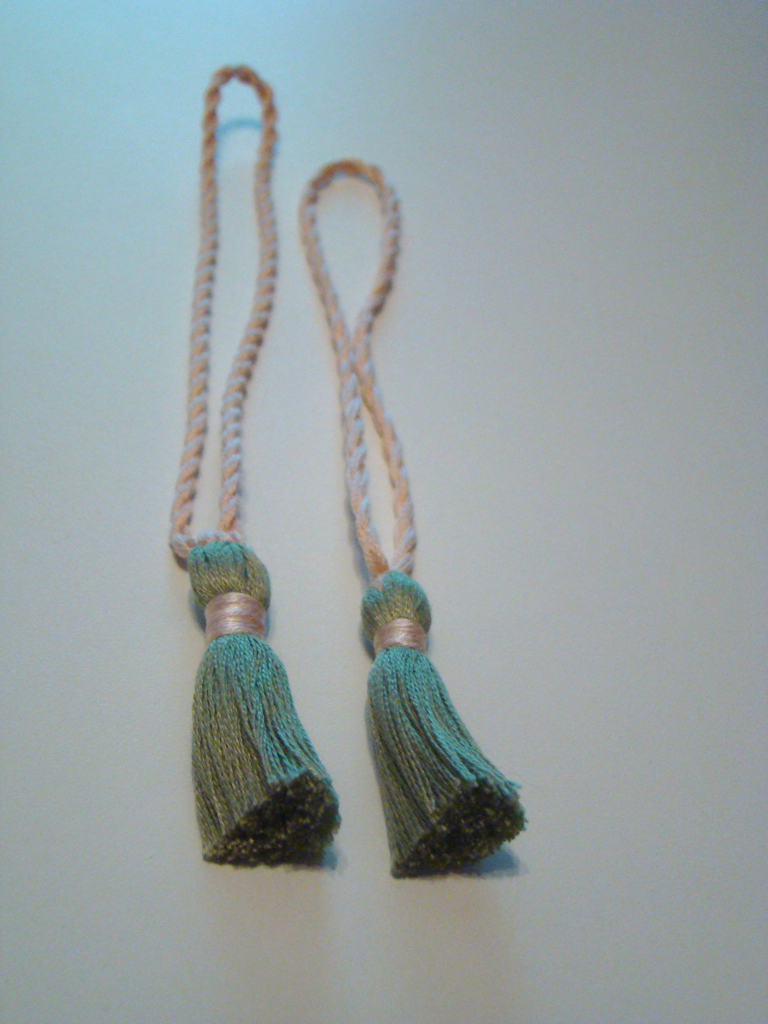This color close-up photograph, possibly taken in studio lighting, features two tassels lying side by side on an underexposed, flat white background that appears slightly gray. The tassels are positioned with their loops pointing towards the top left corner of the image and display light peach, coral-colored cords wrapping around their necks. The tassels themselves are deep green with a soft, flowing texture. Light highlights illuminate the top portions of the cords, while under shadows beneath the tassels add depth to the image. Each tassel features forest green fibers folded and secured with multiple wraps of the coral thread. The left-hand tassel's looped cord is slightly longer than the right, and both are several times longer than the tassels' lengths. The overall image has a subtle blur and gentle shining effect on the cords, accentuated by shadows cast on the background.